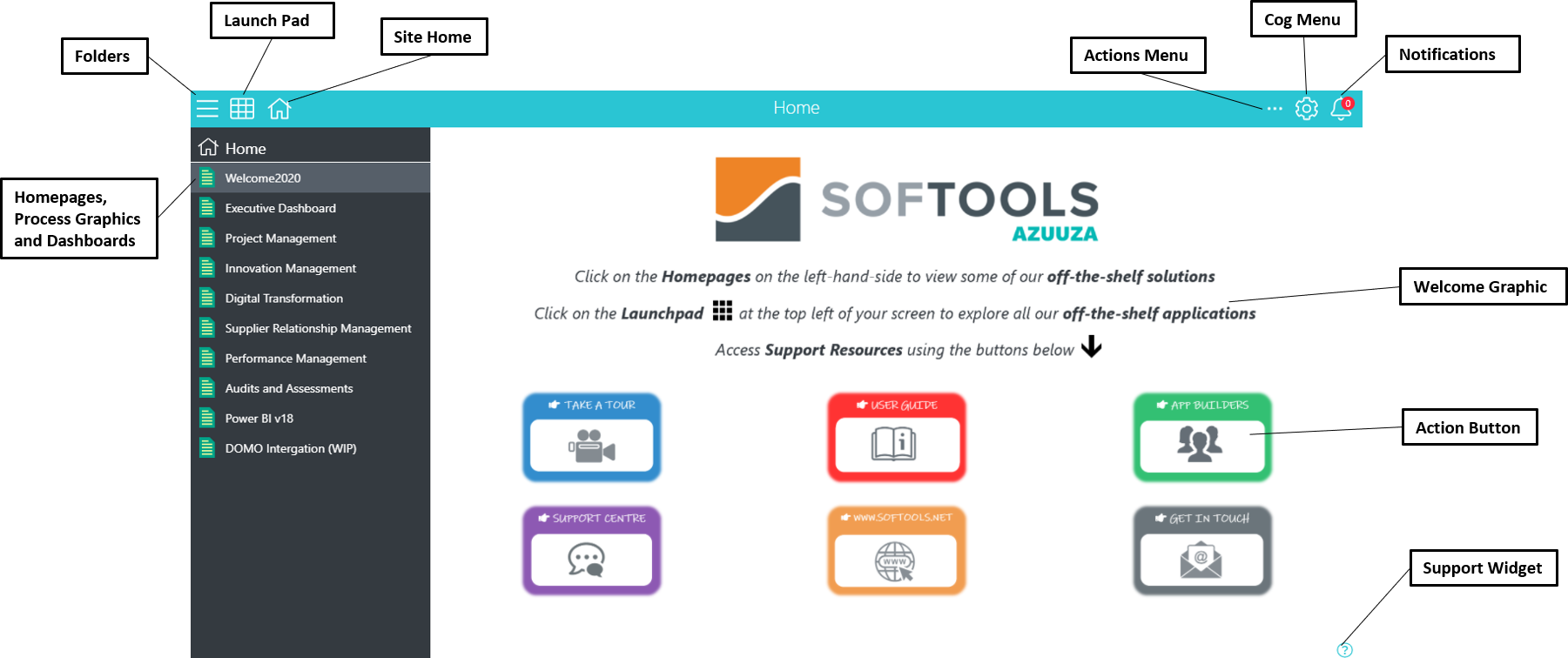The image depicts a website interface labeled "Soft Tools," featuring a detailed navigation bar and various icons.

At the top of the webpage, there is a prominent turquoise strip with white icons:

- **Left Corner**:
  - **Folders Icon**: Represented by three lines stacked vertically, labeled "Folders." The icon is encircled with a black edge, a white background, and black text.
  - **Launch Pad Icon**: Shown as a formation of nine squares organized into a larger square, labeled "Launch Pad."
  - **Home Site Icon**: Illustrated by a house symbol and labeled "Home Site."
  - **Document Icon**: Displayed as a green document with yellow lines, labeled "Home Pages, Process is Graphics, and Dashboard."

- **Right Corner**:
  - **Action Menu Icon**: Three vertical dots labeled "Action Menu."
  - **Cog Menu Icon**: A cogwheel symbol, indicating settings, labeled "Cog Menu."
  - **Notifications Icon**: A bell with a red circle indicating notifications, labeled "Notifications."

On the right side of the turquoise strip, additional elements include:

- **Welcome Graphic Text**: Contains a heading that reads "Welcome Graphic."
- **Action Button**: A button positioned on the front page with the label "Action Button."
- **Support Widget**: Located at the bottom of the page, represented by a question mark within a circle and labeled "Support Widget."

The image captures the structured layout and detailed icons of the "Soft Tools" website interface, providing a comprehensive overview of the navigation elements available to the user.